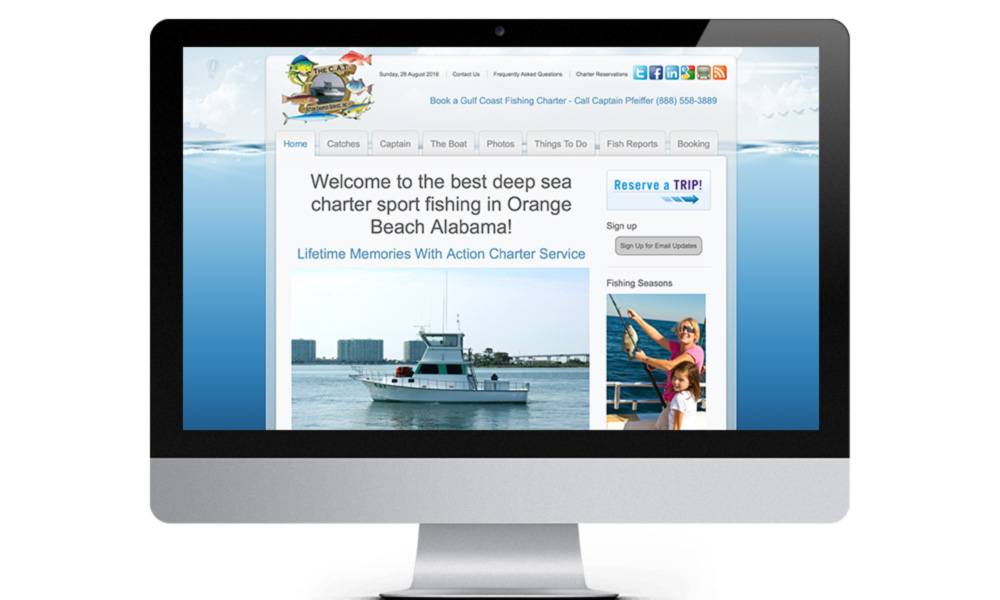In the screenshot displayed in landscape mode, a silver monitor stand is visible at the bottom center, curving inwards to support the monitor from the back. The monitor itself has a prominent black border encompassing its upper left, upper right, lower left, and lower right sections. A silver stripe, matching the stand's color, runs along the bottom of the monitor. Notably, the upper right corner of the black border appears to fade into gray, an anomaly that doesn't typically occur with monitors. A small camera dot is situated at the upper center of this border.

The main content on the screen is a webpage, which could potentially be an app. The background of this page features a scenic image: a sunny sky with clouds at the top, transitioning to ocean waves, and a few birds in the sky on the right side. The ocean itself is a light blue expanse.

The app interface is set against a gray background. In the upper left corner, there is an illustration of a catamaran surrounded by colorful fish, including blue, red, brown, and yellow ones. Several tabs are listed below, reading: "Sunday 28th August 2018 maybe," "Contact Us," "Frequently Asked Questions," and "Change Reservations."

At the upper right corner of the app interface, social media icons for Twitter, Facebook, LinkedIn, and others are displayed. Prominent blue-linked buttons read: "Book a Gulf Coast Fishing Charter" and "Call Captain Pfeiffer 888-558-3889." The active tab, marked in blue, is the "Home Page."